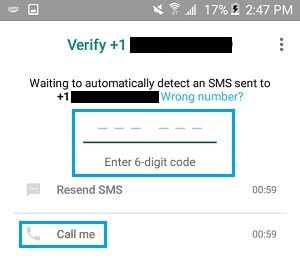In this detailed screenshot, the upper left corner displays a few notification icons, while the upper right corner shows a series of status indicators including the mute icon, Wi-Fi signal icon, network signal bars, and phone battery percentage at 17%. Additionally, an icon indicates that the phone is currently charging, and the time is shown as 2:27 PM. 

The main content of the screenshot features a white background with a grey top section and a black bar across the top. The text reads: "Verify," followed by "Waiting to automatically detect or make some resend to, from number bar." Below that, there is an instruction to "Enter 6 digits code" with options for "Resend SMS" and "Call me." There is also a timer indicating "59 seconds left" for both the "Resend SMS" and "Call me" options.